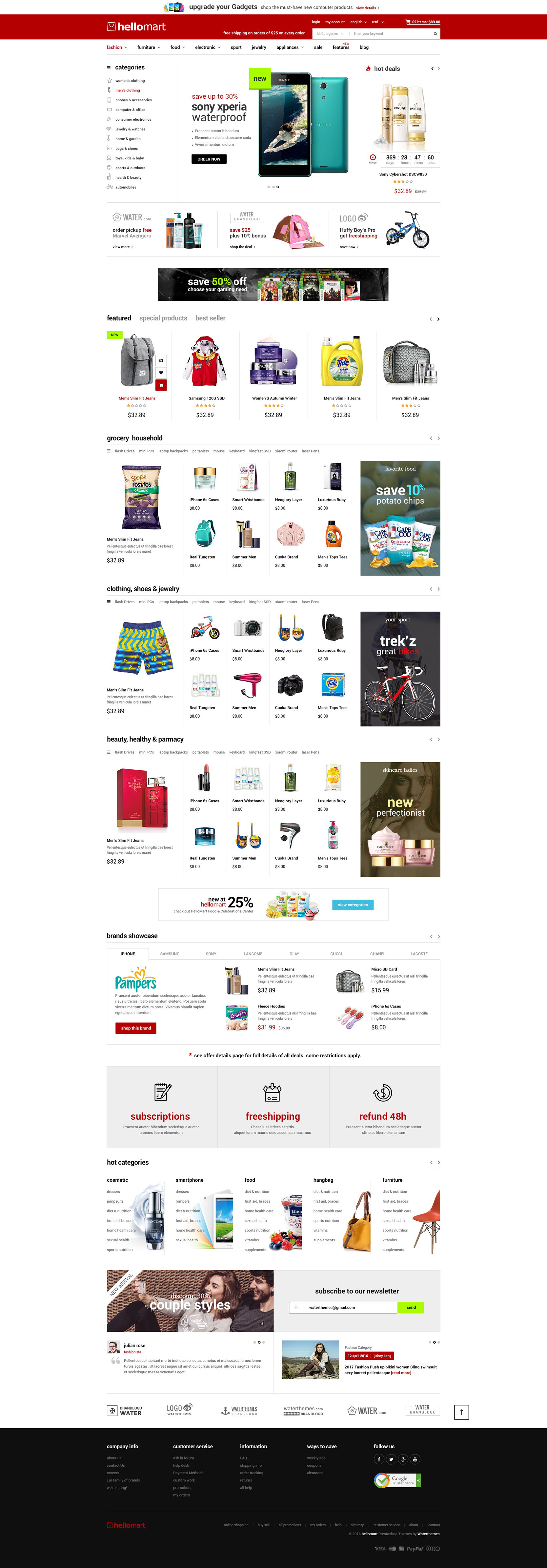The image appears to be a distorted and stretched screenshot from a desktop. The screenshot is of a webpage from a website called Hello Mart, which seems to be an American online store given the visible dollar signs. The website offers a wide range of products, including but not limited to:

- Backpacks
- Perfumes
- Mobile phones, specifically mentioning the Sony Xperia waterproof model
- Bicycles
- Pet food
- Hair products and toiletries
- Camping gear, including a prominently featured tent
- Furniture
- Hair dryers
- Cameras
- Children's jackets
- Car cleaning supplies
- Toiletry bags
- Swimming shorts

The image's quality makes it difficult to read the text clearly, but these categories of goods are discernible.